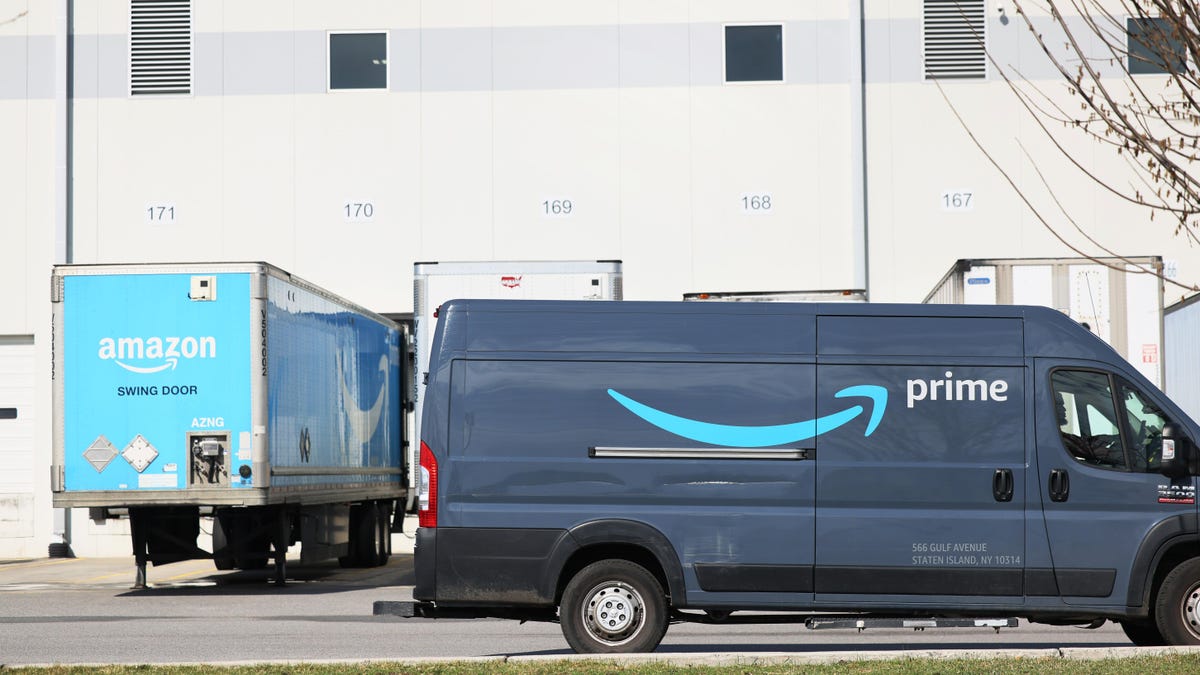The image captures a comprehensive view of an Amazon delivery facility, characterized by multiple semi-truck loading and unloading docks. Specifically, trailers are backed into stalls numbered 167, 168, 169, and 170, while stall 171 remains vacant. Prominently featured in the foreground is a recognizable Amazon Prime delivery van, distinguished by its gray-blue color scheme. Notably, the van has sustained two visible gashes on its side, suggesting it might have slid and collided with an object, potentially during slippery conditions or a minor accident. Despite the damage, the van remains operational, evidenced by the silhouette of a driver inside. The background features a white industrial building with HVAC vents and windows. Lush green grass is visible at the bottom edge of the image, framing the scene. This detailed snapshot illustrates the daily operations and logistical setup of an Amazon loading, unloading, and sorting facility.